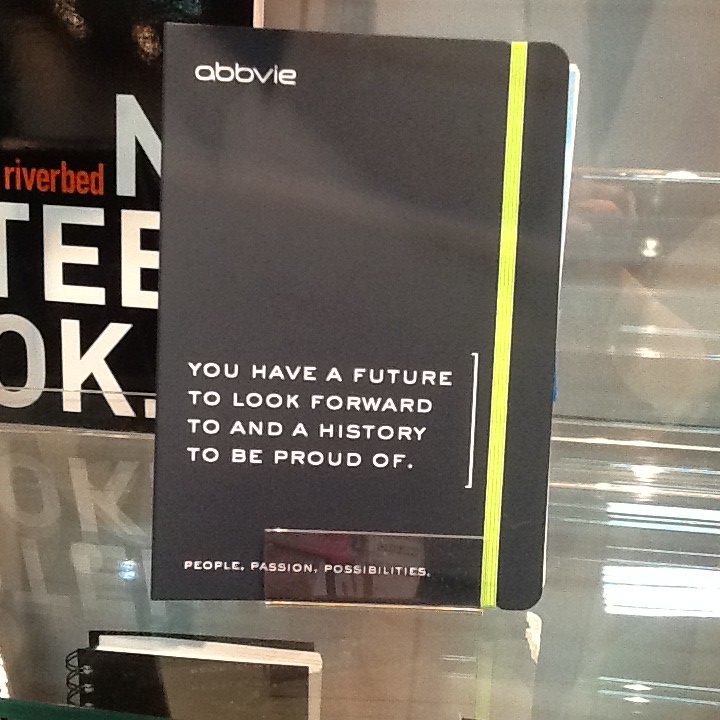This image captures a planner book from the brand ABBVIE, prominently displayed on a shelf or possibly a desk, encased in a translucent, rectangular holder. The cover is primarily black with a notable vertical yellow band on the right side. In white capital letters on the upper left corner, the name "ABBVIE" is displayed, and further down the cover are the inspirational words: "You have a future to look forward to and a history to be proud of." At the very bottom, the phrases "People, Passion, Possibilities" are highlighted. The background is blurred, revealing a barely discernible sign with the word "riverbed" in small red letters and only a partial view of an adjacent notebook. The overall scene suggests a minimalistic and professional display with a color scheme dominated by black, gray, and gold.